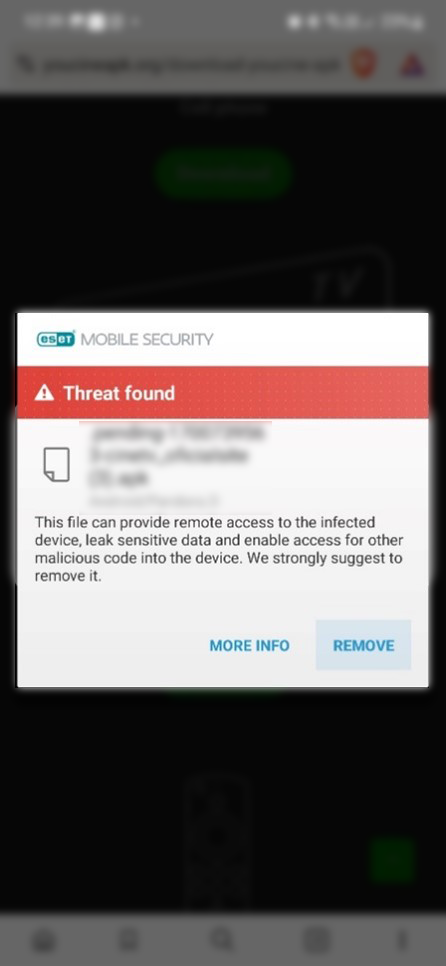This image, captured from a phone screen, features a blurred background with most elements obscure and indistinct. The top portion of the phone is lighter in color, and a smaller horizontal section at the bottom, though blurred, reveals some partially obscured icons. Dominating the image is a large black section, which encompasses the middle of the screen. At the center of the black area lies a blurred horizontal green oval.

Central to the image is a white pop-up notification with the title "Mobile Security" in light gray font, accompanied by a small logo. Below the title, there's a prominent coral-colored horizontal rectangle containing a white triangle symbol with an exclamation mark, followed by the warning text "Threat Found" in white font. The subsequent details under this warning are partially blurred but still readable: "This file can provide remote access to the infected device, leak sensitive data and enable access for other malicious code into the device. We strongly suggest to remove it."

At the bottom of the pop-up, two small horizontal buttons are visible. The first button, with a white background, contains the text "MORE INFO" in capital letters with turquoise font. Adjacent to it, the second button is light blue with the text "REMOVE" in capital letters, also in turquoise font.